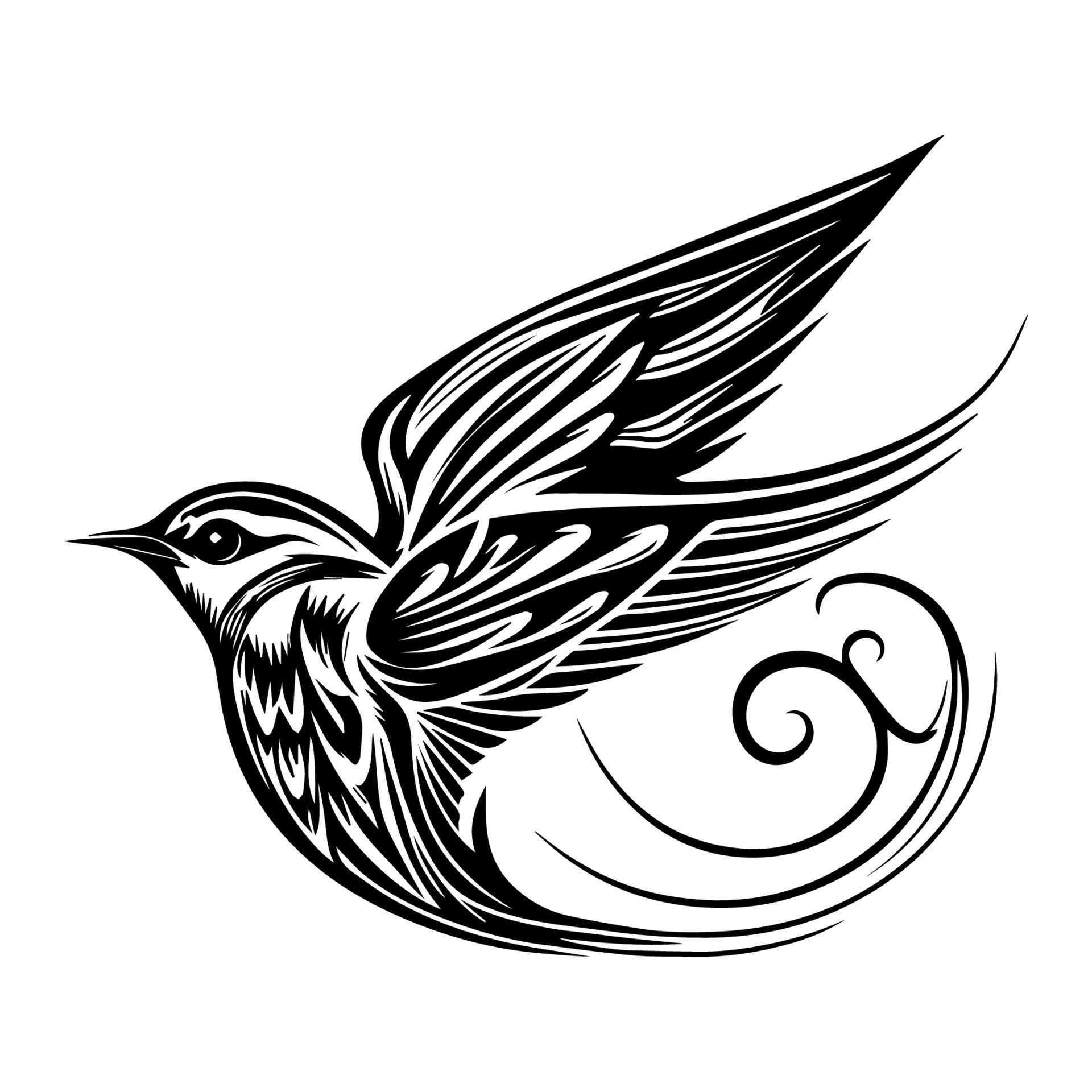This detailed drawing on a stark white background depicts a fanciful bird, resembling a hummingbird in profile, facing left. Rendered in black and white, the bird has an elongated, sharp beak and a prominent black eye. Its wings are extended to the right, characterized by graceful, tapered feathers. Notably, instead of a realistic tail, the illustration features a flowing black swirl, suggesting motion and flight. The bird's breast showcases intricate feather details, further enhancing the elegant linework. This stylized image, reminiscent of a tattoo design, captures the essence of a bird in mid-flight, emphasizing its dynamic and artistic form rather than anatomical accuracy.